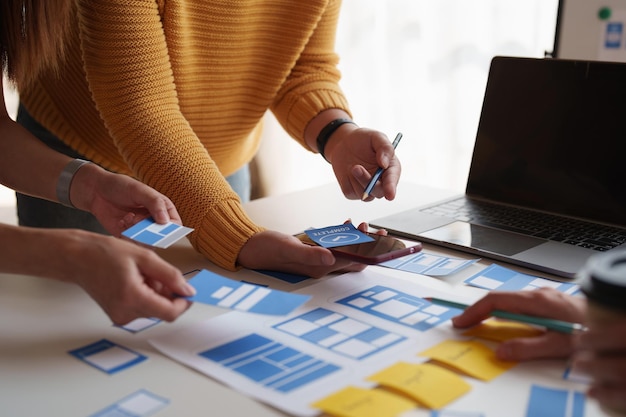Indoor color close-up photograph showcasing a collaborative Kanban scheduling session. The scene is set in a generic office environment with a large table occupying most of the frame. On the table, there are various task cards, blue and yellow post-it notes, and a white sheet of paper with blue patterns, possibly scheduling ideas. Three people are engaged in organizing the tasks: one person, only visible by their outstretched hands, is in the top left with an unseen face, another person is partially visible on the right side of the table wearing a mustard yellow sweater, holding a card in her left hand and a blue pencil, while the right hand holds a cell phone with a blue card on it. In the lower right corner, another hand is seen holding a green pencil. A MacBook with a black screen is positioned in the upper right corner of the table. The casual attire of the individuals suggests a relaxed working atmosphere, possibly among marketing specialists or office workers involved in a project or process organization session.